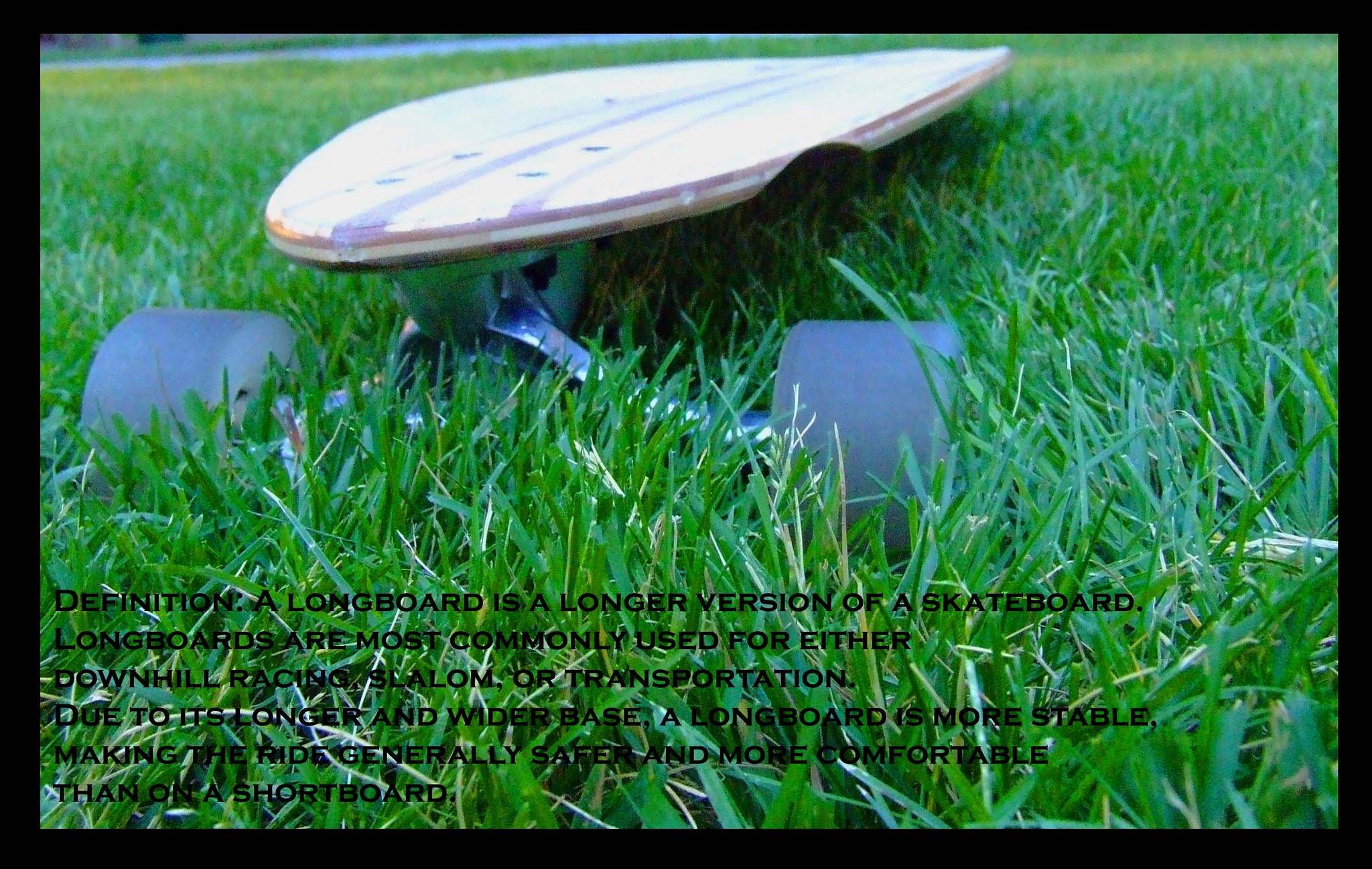This vibrant outdoor photograph framed by a black border captures an orangish-yellow longboard with a red stripe resting amidst tall, lush, green grass, appearing to be around four or five inches high. Taken from a low angle, the perspective focuses on the front part of the longboard, highlighting its gray wheels attached to the metal trucks. The back wheels are not visible. Black text printed on the grass near the bottom left corner reads: "definition: A longboard is a longer version of a skateboard. Longboards are most commonly used for either downhill racing, slalom, or transportation. Due to its longer and wider base, a longboard is more stable, making the ride generally safer and more comfortable than on a shortboard." The scene suggests a sunny day, emphasizing the longboard's details and the grass's vibrant hue.